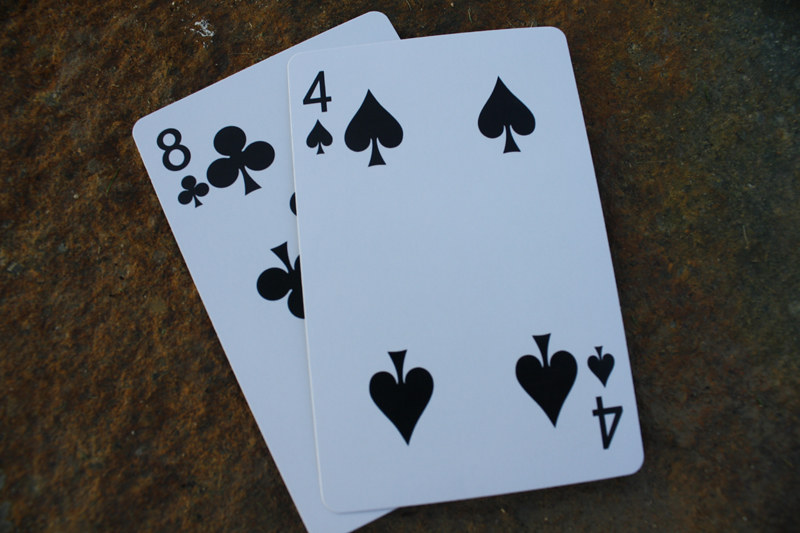This is a highly detailed close-up photograph of two playing cards from a deck, placed against a blurry background that showcases a blend of brown, yellow, and greenish hues, suggesting it could be a floor or a table. The focus is sharp on the cards, capturing their intricate details. The bottom card in the image is the eight of spades. The eight is prominently displayed in the top left and bottom right corners of the card, with a small spade symbol adjacent to each number. Additionally, two larger spade symbols are partially visible, one near the upper center and the other, upside down, near the lower center of the card. Overlaying the eight of spades at an angle is the four of clubs. This card is fully visible, with the number four displayed in the top left and bottom right corners— the latter being upside down. Each number is accompanied by a small club symbol. The card also features four large club symbols arranged with two at the top and two at the bottom, perfectly symmetrically aligned.